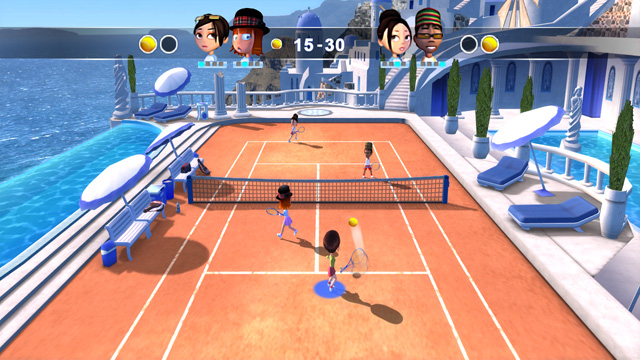A vivid scene from a video game showcases an intense tennis match on a brown court bearing white lines that delineate its sections. On either side of the net, which divides the court down the middle, stand two teams, each comprising two players. The left team features two female characters, while the right team consists of one female and one male character. A yellow tennis ball, trailed by a white stream, is captured mid-air during the rally. Both sides of the net have benches shaded by cloth canopies, providing respite for the players. Adjacent to the court are swimming pools on either side, adding a touch of luxury to the setting. Stairs ascend from the foreground, leading to different elevations within the game's environment. The scoreboard at the top of the screen displays a current score of 15-30, accompanied by a black and yellow ball icon next to each team.